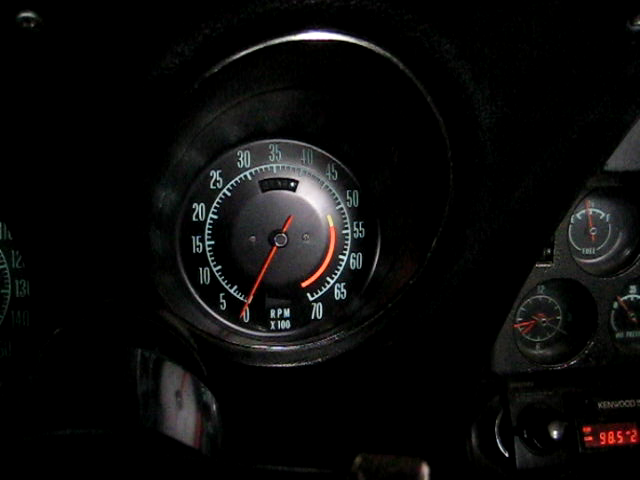The image depicts a portion of a car dashboard with a primary focus on a circular RPM gauge against a dark black background. The central dial prominently features the letters "RPM" at the bottom, indicating its purpose of measuring rotations per minute. The gauge spans from 0 on the left to 70 on the right, with white numerical increments marked every 5 units. A red pointer, fixed at the center, indicates the current RPM measurement.

To the right of the main RPM gauge, there are three smaller dials, each with red hands and white numerical markers, similar to a clock. The precise function of these dials remains unclear due to the lack of visible labeling. In the bottom right of the image, a small rectangular display shows the number "98.5" and is accompanied by a black knob on the left side, resembling a car’s radio interface. No additional text is present in the image.